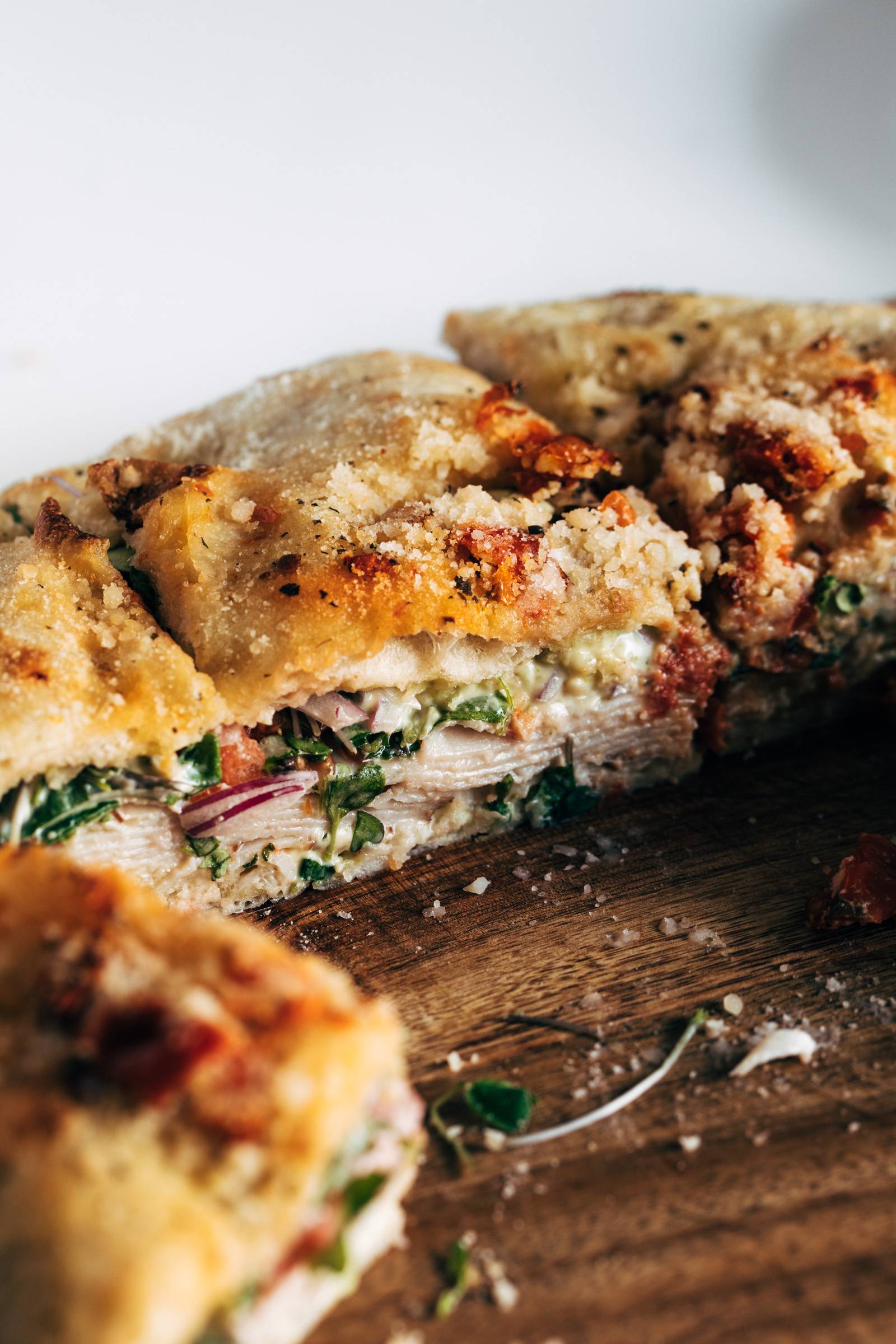This close-up digital photograph showcases a delicious, multi-layered dish resembling a lasagna. Each piece is square and features a golden-brown, caramelized, and crusty top layer with a dusting of cheese. Below the crispy top, we see layers of flaky off-white crust, vibrant red onions, and green herbs, possibly diced spinach. The interior reveals layers of meat and vegetables meticulously assembled to create a hearty meal. The dish is set on a dark, richly textured wooden cutting board, which is scattered with crumbs and small pieces of green vegetables. The photo composition includes four pieces of the dish, with one piece being slightly pulled out toward the lower left corner, blurring into the foreground. The top portion of the image is a blurred, whitish-gray background that contrasts with the warm, rich colors of the food.